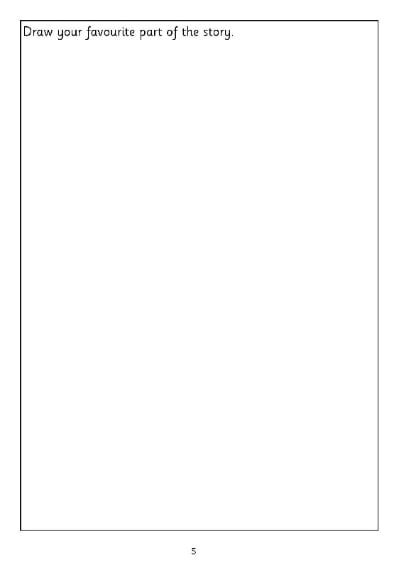The image is a simple layout presented on an 8.5 by 11 inch paper. In the top-left corner, there is a line of text in a casual font reminiscent of Comic Sans, albeit slightly more formal. The text, which is in black, reads: "Draw your favorite part of the story." The first letter "D" is capitalized and the phrase ends with a period. This text is framed within a black rectangular border that surrounds the entire page, although the color of the border varies slightly. The left and top edges of the border are a more defined black, while the right and bottom edges appear in a softer, grayer shade. At the very bottom of the page, just outside the main border, the number "5" is written, indicating a page number. Other than these elements, the image contains no additional content or details.